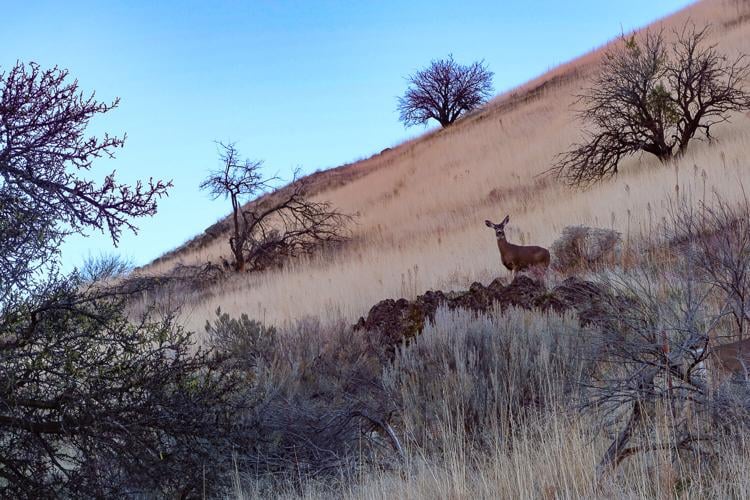A lone doe stands perched atop a rocky outcrop on a steep, hilly terrain, covered in tall, dried grass that has taken on a light tan, wheat-like hue. The hill slopes from the lower left to the upper right, dotted intermittently with leafless shrubs and stubby, brown-branch trees indicating a fall or late autumn setting. The clear blue sky above adds a tranquil backdrop to the scene. The deer, with its dark brown fur and white markings on its ears, gazes curiously toward the camera, perhaps wary of the photographer's presence. Another deer may be slightly visible to the right, blending seamlessly with the sparse vegetation and rugged landscape. The entire scene is bathed in natural daylight, bringing out the earthy tones and textures of this serene, outdoor nature shot.